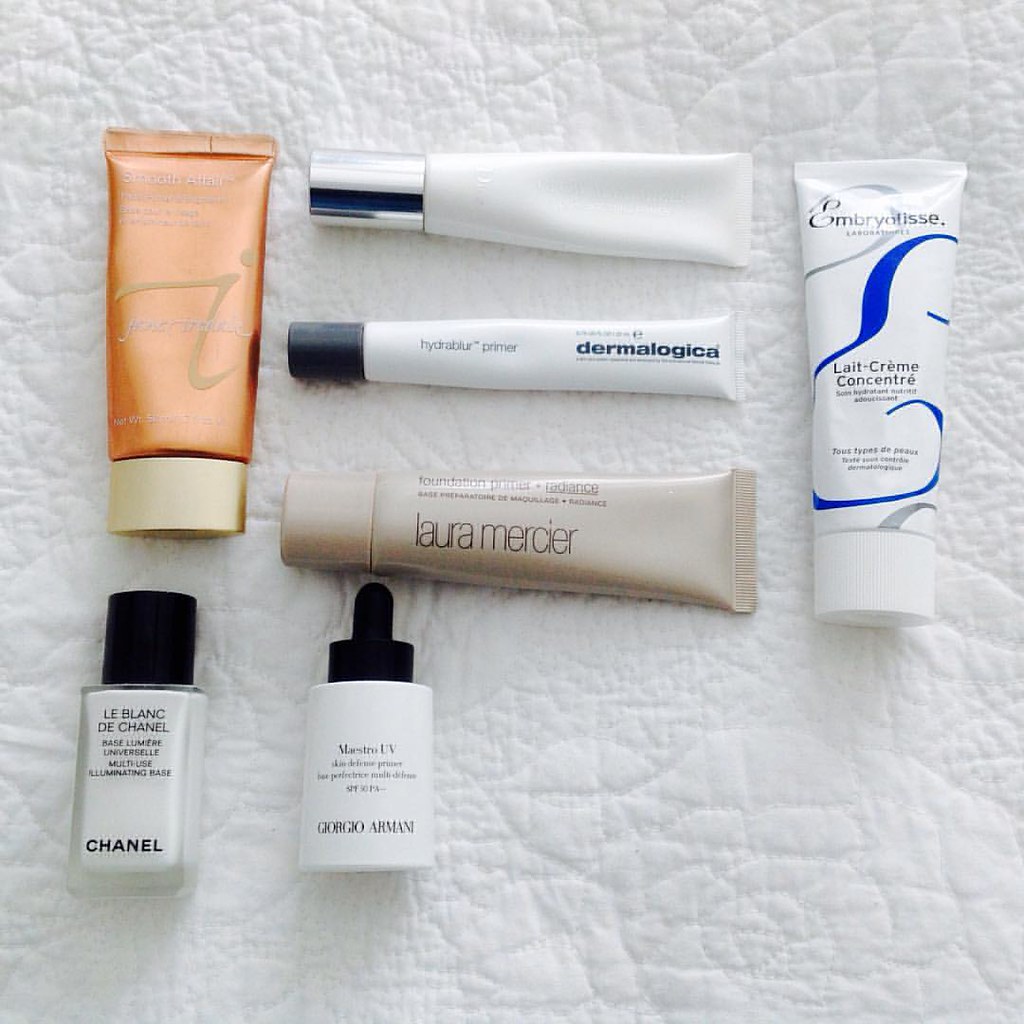The square, well-lit, and crisp color photograph features a display of various skincare items carefully laid out on a textured white background that mimics the appearance of alligator skin, although it might be quilted cotton fabric. 

In the top left corner is a coppery-orange squeeze tube with a screw-on cap, resting upside down, its details obscured by glare. Below it, in the bottom left, is a small, rectangular bottle with a black screw-on top containing a white substance. The label reads "Le Blanc de Chanel" with "Chanel" prominently displayed at the bottom.

Centrally located are three squeeze tubes lying side by side. The top tube is white with a chrome-colored screw-on cap. The middle tube, also white but slimmer, has a black screw-on cap and is labeled "Dermalogica" with "Hya-something Primer" written on it. The third tube, in a tan hue with a matching cap, is labeled "Laura Mercier."

Adjacent to the Chanel bottle is a short, white Giorgio Armani bottle featuring an eyedropper bulb screw-on top, its exact contents illegible due to small print. Lastly, a larger squeeze tube marked "Embryolisse" in blue script occupies the right side of the frame. The label reads "Le Crème Concentré," indicating it as a moisturizing lotion or cream.